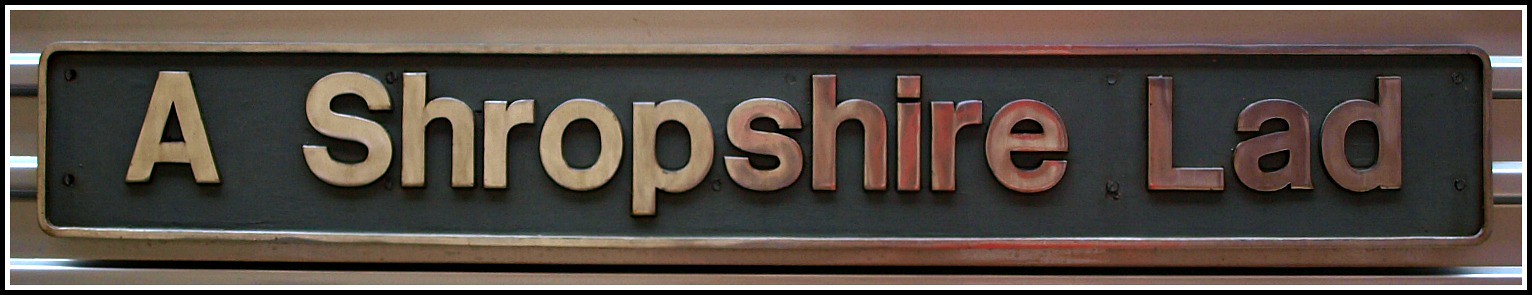The image showcases a meticulously crafted sign that reads "A Shropshire Lad." The sign features an elegant black metal background, accentuated by silver lettering and a polished silver frame. It is securely mounted on two horizontal silver metal bars, with an additional horizontal silver bar visible just below the sign. The backdrop is a warm, brownish-tan surface, providing a contrasting setting for the sign. The sign itself is adorned with several rivets—one in each of the four corners and another strategically placed between the words "Shropshire" and "Lad." This detailed setup highlights the sign's refined yet robust design.